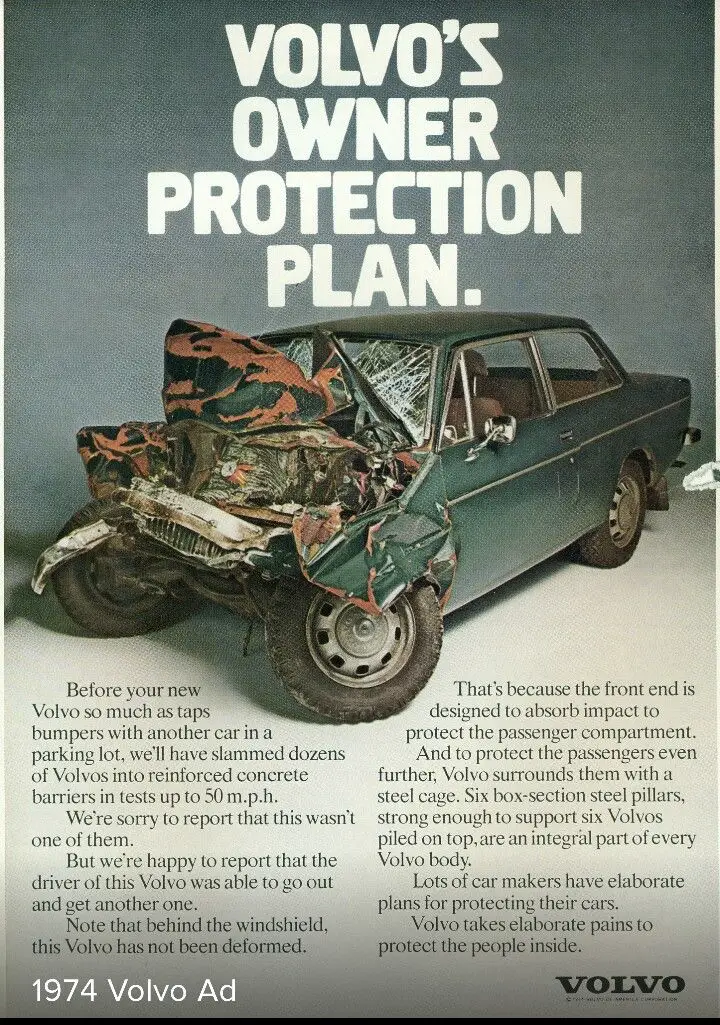The image is a 1974 portrait-mode Volvo advertisement with a gray gradient background that features a smashed up green Volvo car. The headline at the top in white text reads "Volvo's Owner Protection Plan." Beneath it, there's an extensive narrative detailing Volvo's rigorous safety testing, which includes slamming dozens of cars into reinforced concrete barriers at speeds up to 50 miles per hour. The front end of the showcased Volvo is severely mangled with a shattered windshield, although the passenger compartment remains intact, emphasizing the car's ability to absorb impact to protect its occupants. This resilience is attributed to the inclusion of a steel cage and six box section steel pillars, which are strong enough to support six Volvos piled on top. At the bottom left corner, it notes "1974 Volvo ad," and the bottom right corner features the Volvo logo in dark text. The ad conveys that although the car depicted wasn't one from their tests, the driver nonetheless walked away safely and was able to get another Volvo, underscoring the brand's commitment to passenger safety over vehicle preservation.